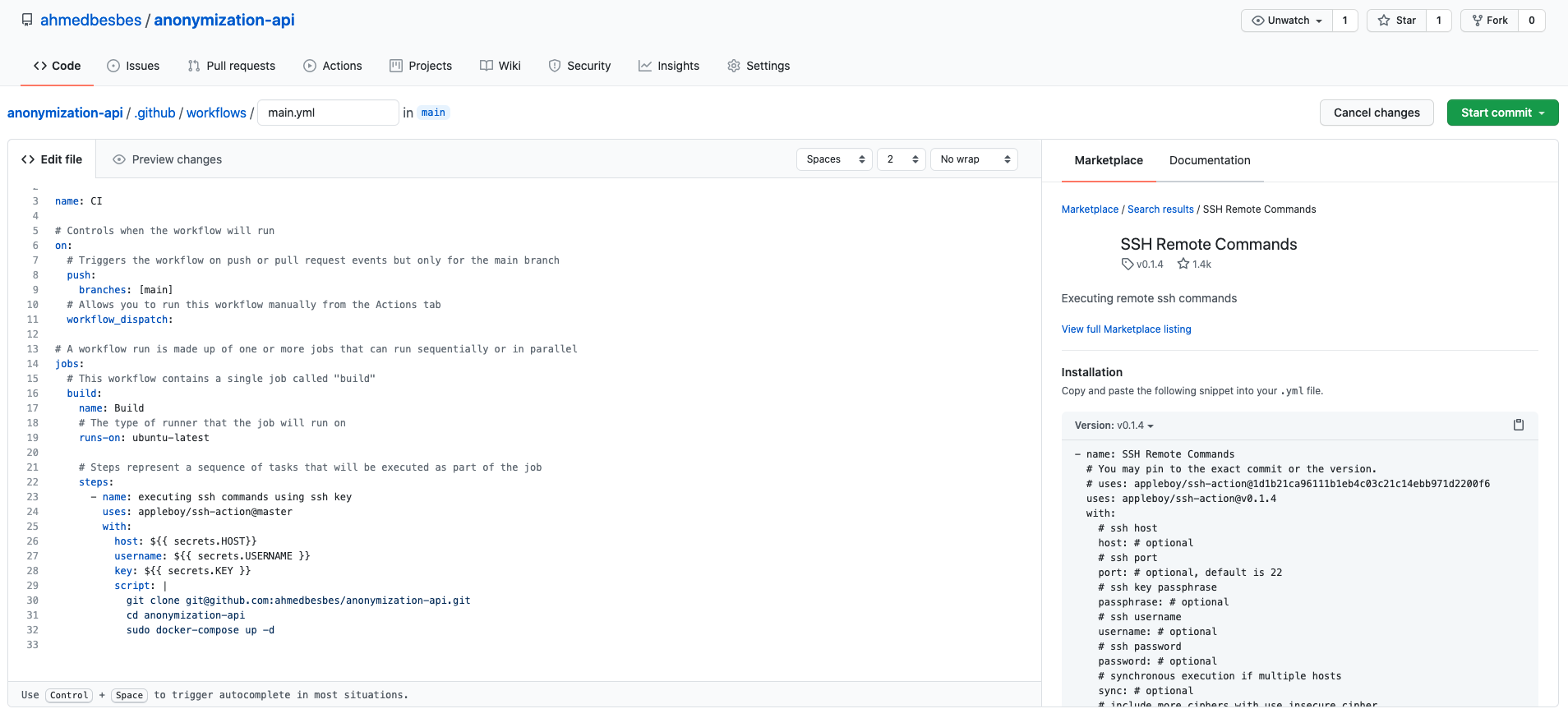The webpage exhibits a layout typical of a GitHub repository, albeit with several blurred and small text elements. In the upper left corner, the page displays the repository name "AHMEDBESBES/anonymization/API" in blue text. Below it, the word "code" is prominently displayed in black with a red underline, indicating the active tab. Adjacent to this is a series of navigation tabs for different repository functionalities: Issues, Pull Requests, Actions, Projects, Wiki, Security, Insights, and Settings.

Below the navigation tabs, the exact path "anonymization/API/GIHub/workflows" is marked in blue, suggesting a deeper navigation path within the repository. There's an icon resembling a speech bubble with text too blurred to read. Further below, options such as "edit file" and "preview changes" are available, hinting at current file editing modes.

The page features drop-down tabs with labels like "spaces" and "no wrap." Displayed code alternates between blue and black, presumably indicating syntax highlighting, with line numbers ranging from 1 to 33 along the left margin. 

In the upper right corner, there is a box labeled "cancel changes" next to a green box partially visible with the word "start" at the beginning. Further down the page, under a red-underlined “marketplace” in black text is followed by “documentation.” Below this section, the term “SSH remote commands” appears, leading into more code.

Overall, the webpage provides a glimpse into the structure and features of a GitHub repository, albeit with some details blurred and challenging to read.